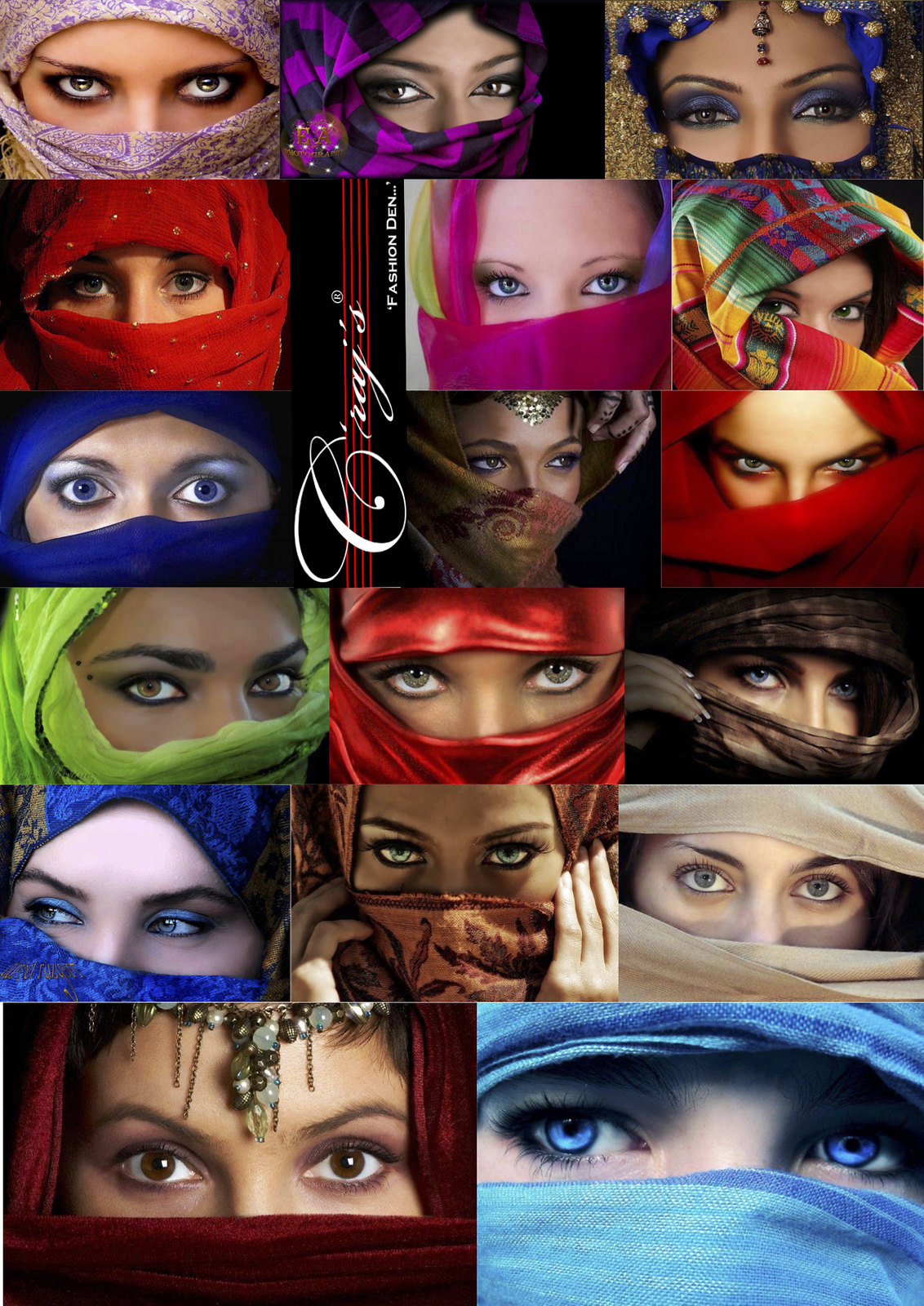The image is a detailed photo montage showcasing the eyes of women wearing vibrant, colorful veils. The women have their faces mostly covered with the scarves, leaving only their eyes and eyebrows visible. These scarves come in various colors, such as maroon, lime green, red, blue, pink, purple, black, and even some with patterns like paisley. Some women feature intricate makeup around their eyes, while others have a more natural look. In several cases, the women also wear decorative headbands or tiaras with beads, adding to the visual interest. The largest and most striking image at the bottom shows a woman with piercing bright blue eyes, her head wrapped in a matching blue scarf. In another standout image at the bottom left, a woman wears a maroon scarf with a jeweled headband. This montage appears to be for a fashion ad, possibly for Grey's Fashion Den, reflecting a Middle Eastern style that emphasizes the beauty and expressiveness of the eyes.